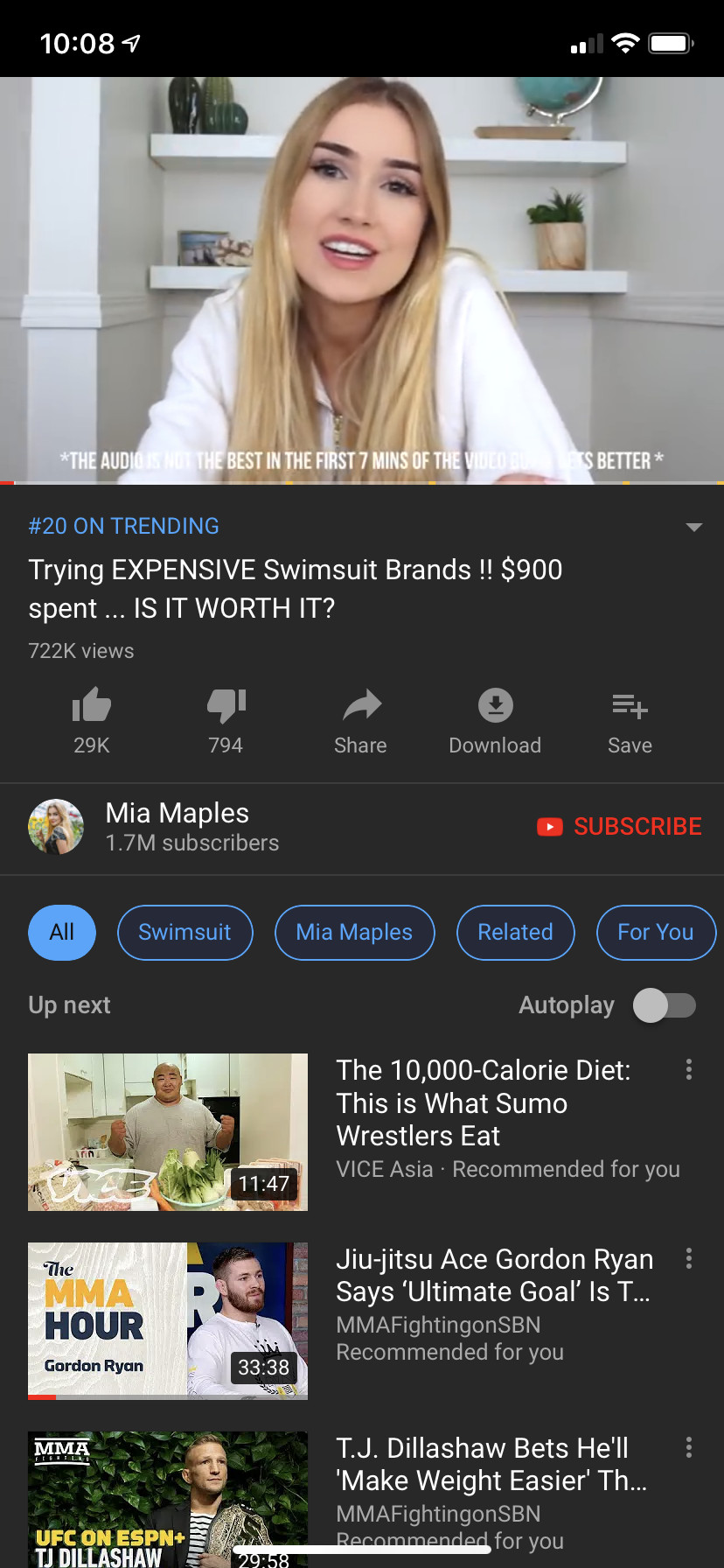The image is a screenshot taken from the mobile application YouTube, captured at 10:08 AM. In the top left corner, the time is displayed, while the top right corner shows indicators for battery life, Wi-Fi strength, and cellular signal strength, confirming that the screenshot is from a mobile device.

At the top of the screenshot is a video thumbnail featuring a woman with blonde hair wearing a white shirt, appearing to speak directly to the viewer. The video's title, "Try an Expensive Swimsuit Brands, $900 Spent, Is It Worth It?", is displayed below the thumbnail. The video is uploaded by Mia Maples, who has 1.7 million subscribers. The video has garnered 29,000 likes and 794 dislikes. Beneath the video title are options to share, download, and save the video.

At the bottom of the screenshot are four suggested videos, displayed as a playlist. The titles of these videos are as follows: "The 10,000 Calorie Diet," "Jiu-Jitsu Escorted Ryan Says Ultimate Goal," and "TJ Dillashaw Bets He'll Make Weight Easier."

The application is set to dark mode, with the background in shades of dark black and grey.